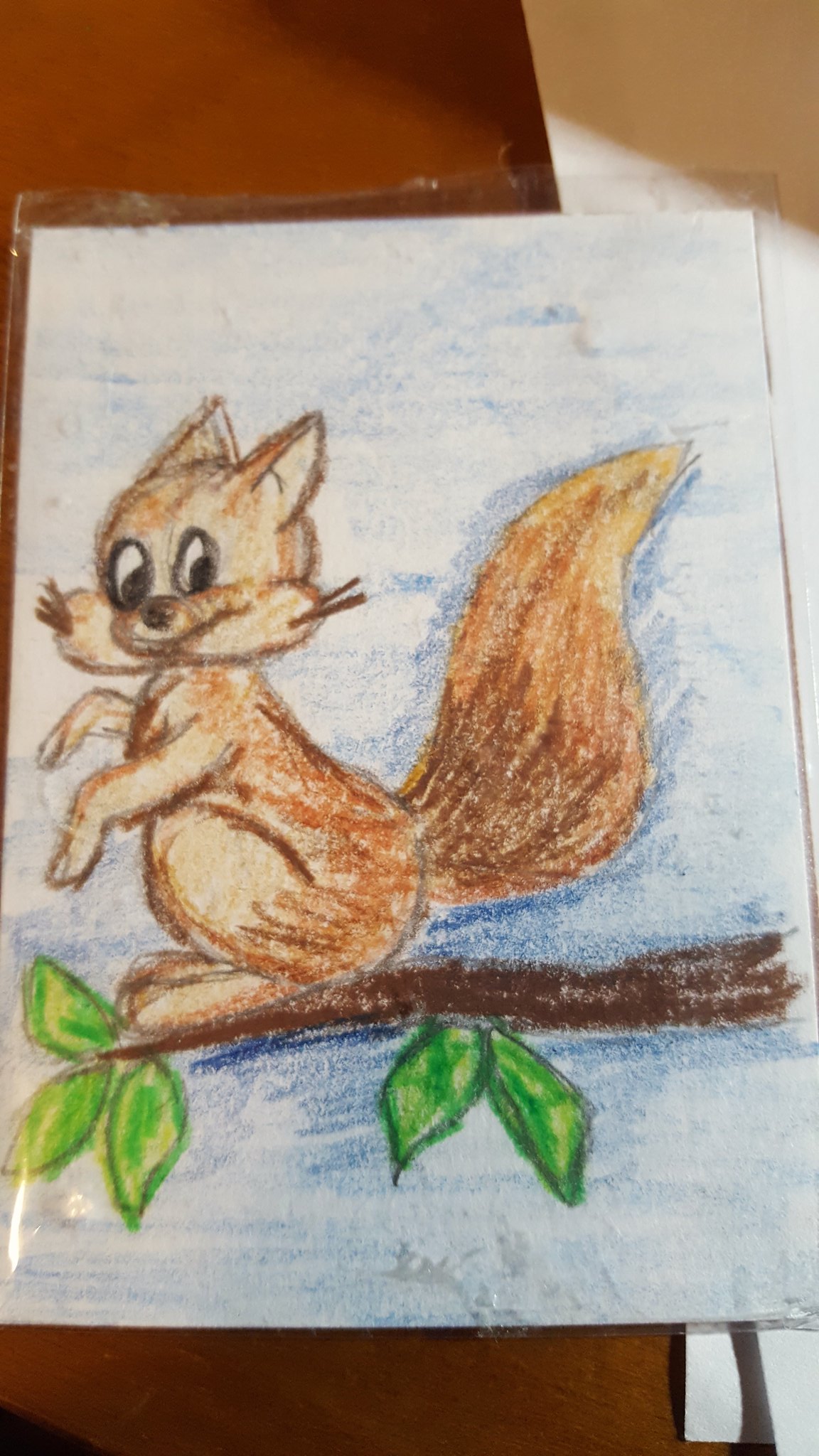This overhead photograph features a crayon drawing on a piece of laminated paper. The lamination is evident from the visible plastic edges at the top and sides, as well as a noticeable glare in the bottom left corner. The image rests on a dark wooden surface, contrasting with the bright colors of the drawing itself. The artwork depicts a cartoon squirrel perched on the very end of a branch that extends to the left side of the paper. The branch is adorned with vibrant green leaves. The squirrel, characterized by its long, bushy tail, gazes directly at the viewer with expressive, cartoonish eyes, adding a whimsical charm to the scene.